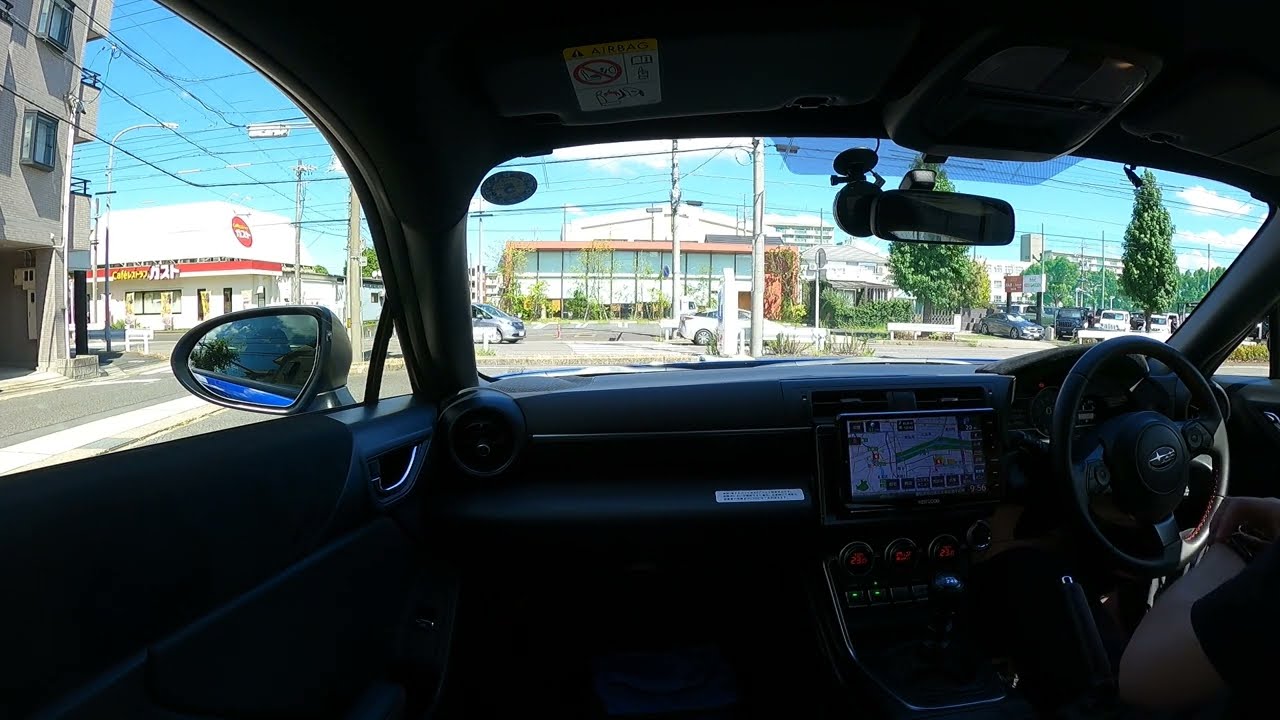This wide rectangular photograph captures the detailed interior of a black sports car from the perspective of the front seat. The streamlined dashboard features a small, specialized steering wheel on the right side, adorned with a central silver star-shaped emblem. Adjacent to the steering wheel is a GPS tablet. Towards the bottom right, the driver's elbows are partially visible. 

Through the car's windshield and side windows, an urban streetscape unfolds. Dominating the view in front is a multicolored building in green, orange, and gray hues, situated behind a horizontal gray road. To its right, several lush green trees are visible under a partly cloudy blue sky. On the left-hand side, the view extends to a side mirror and what appears to be a gray, multi-storied apartment building. Further to the left, parked vehicles and a brick building with many windows are also visible. A white truck is stationed directly in front of the main building, contributing to the bustling street scene.